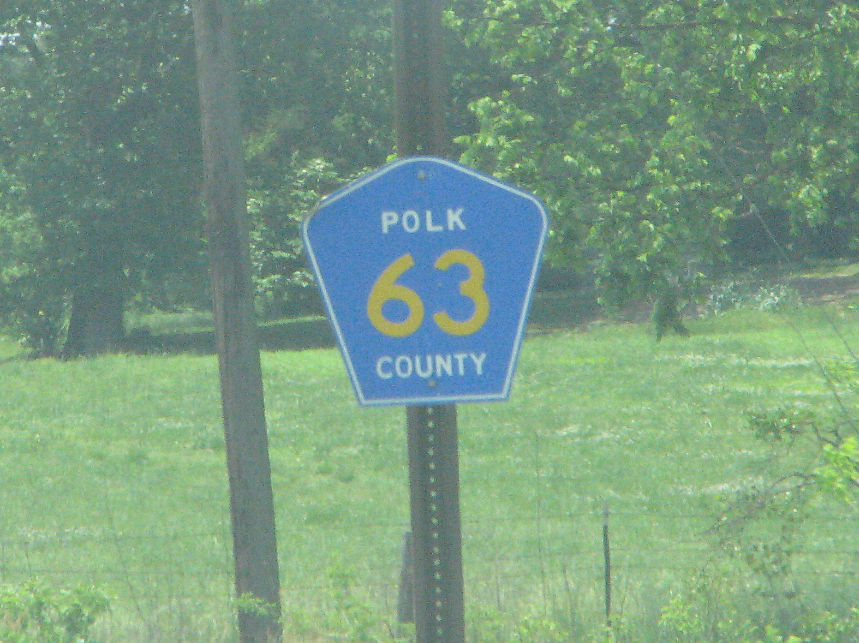A daytime photograph capturing an outdoor scene with a lush, green grassy field interspersed with patches of white flowers in the background. The field is bordered by an array of verdant trees, characterized by their dark trunks and dense foliage. In front of the field, a sturdy metal fence stands as a barrier. Prominently positioned near the foreground is a large wooden telephone pole. Closer to the frame, a road sign is mounted on a metal post. The sign, blue with a white outline, reads "Polk County" in white letters, with the numbers "6" and "3" displayed in yellow between the words. Surrounding the base of the post, green weeds and the branches of small trees add a touch of untamed nature to the scene.